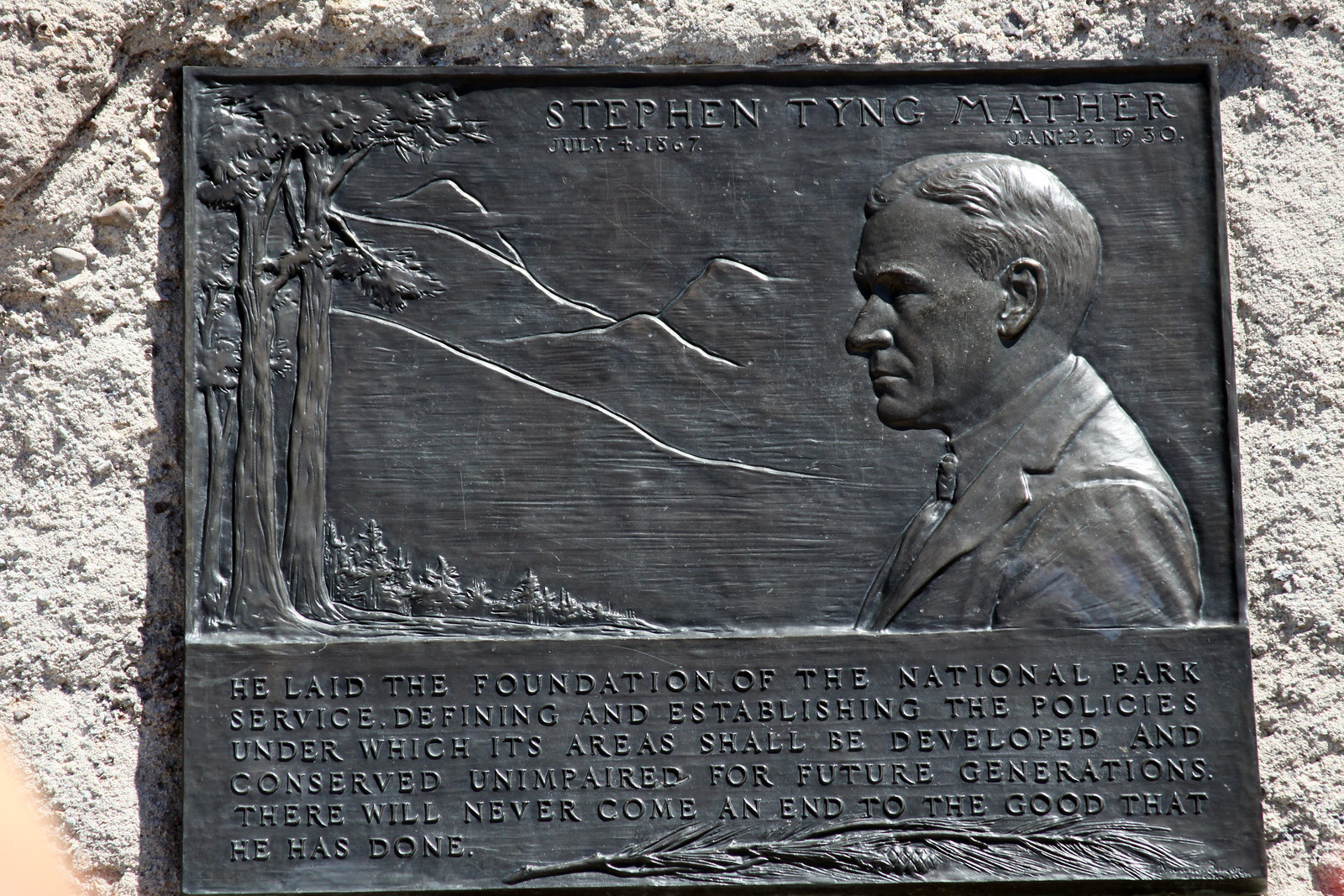The image is a detailed photograph of a dark metal placard, likely brass or silver, set into a grainy white and gray stone wall. The placard features an etched profile of a clean-shaven man with close-cropped hair, dressed in a business suit, and looking off to the left. The inscription at the top reads, "Stephen Tyng Mather, July 4, 1867 to January 22, 1930." Surrounding the man's profile are etched depictions of trees and mountains. Below the image, the placard commemorates Stephen Tyng Mather's significant contributions with the text: "He laid the foundation of the National Park Service, defining and establishing the policies under which its areas shall be developed and conserved unimpaired for future generations. There will never come an end to the good that he has done."